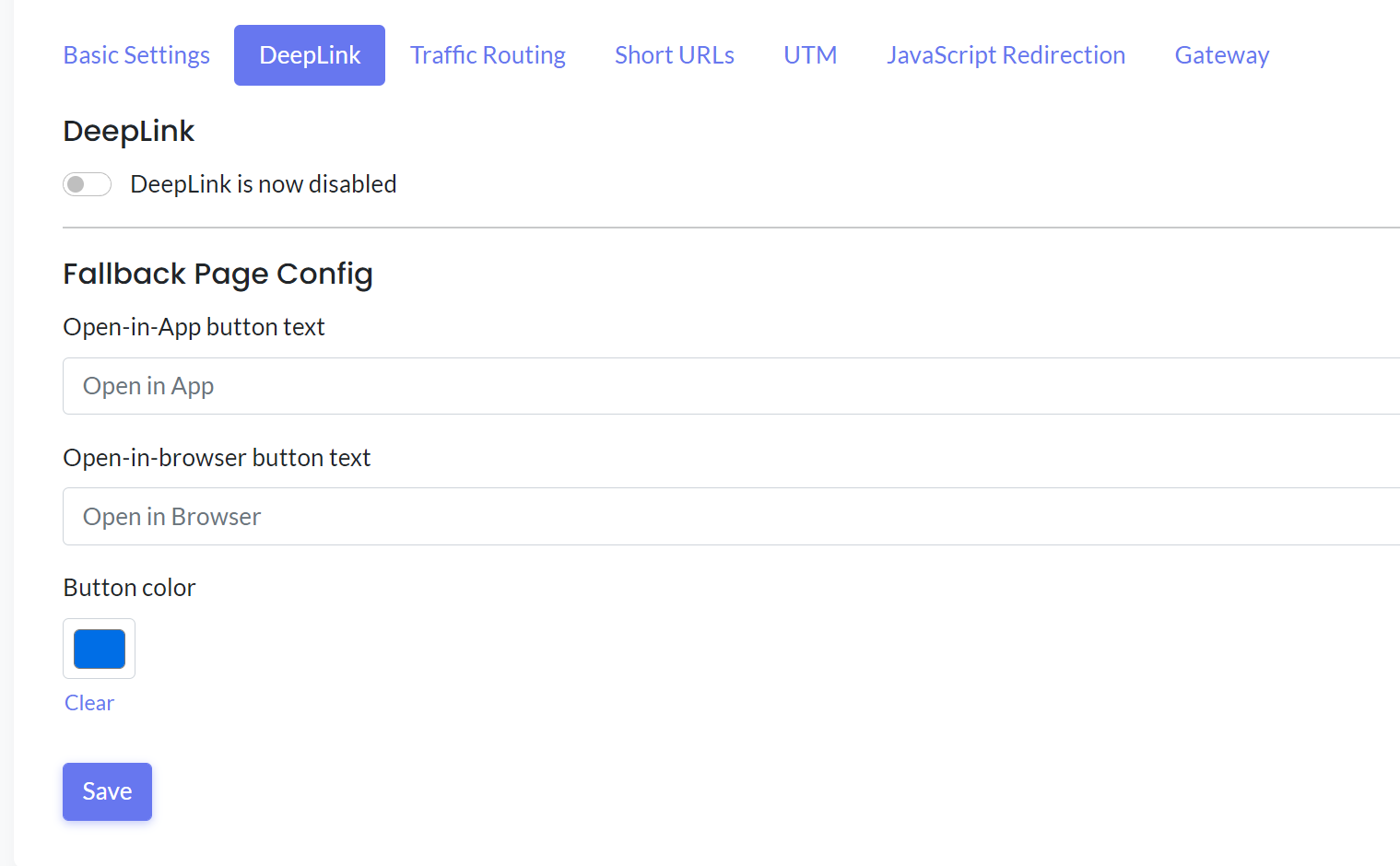The image displays a laptop screen with a settings dialog box open, set against a clean white background. The title of the current settings category, "Deep Link," is prominently highlighted with a blue background and white text, indicating it is the active selection. Within the blue-bordered box labeled "Deep Link," the title "deep link" appears in large black font. Below it, a slider button indicating the status of the deep link is shown in the off position, slid to the left, and labeled "Disabled."

A horizontal line separates this section from the "Fallback Page Config" settings, which is presented in bold text. Below this heading, two options are available: "Open in app button text" with an associated input box labeled "Open in app," and "Open in browser button text" with another input box labeled "Open in browser." The "Open in browser" setting details the button color as blue, complemented by a "Clear" option depicted as a hyperlink.

At the bottom of the dialog box, a "Save" button, also in blue, finalizes any changes. Surrounding these active elements, the interface offers additional settings options such as "Traffic Routing," "Short URLs," "UTM," "JavaScript," "JavaScript Redirection," and "Gateway," all in blue text. These options are inactive but selectable, contrasting with the active "Deep Link" setting that has white text on a blue background. The overall design is straightforward, with consistent font usage except for slightly larger headings that demarcate different sections.